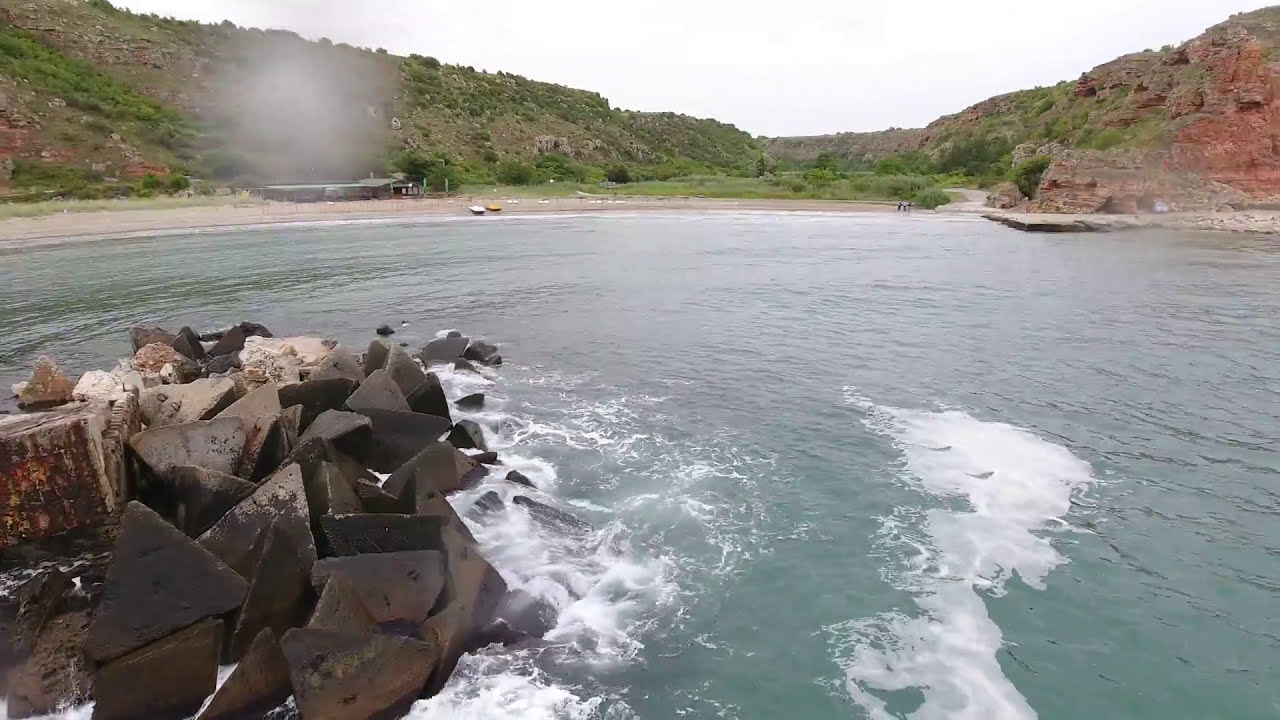A horizontal daytime photograph shows a expansive greenish-blue body of water, likely a lake. The water occupies the bottom two-thirds of the image and is choppy, with frothy white waves, particularly in the foreground near a rocky outcrop on the left. These dark brown and light brown rocks, some with sharp, pyramid-like edges, rise dramatically from the water. Besides the rocks, there are also logs partially submerged, adding texture to the scene. The background showcases a beach with light-brown sand, dotted with a few buildings, one of which is brown but partially obscured by an obstruction on the camera lens. Resting on the sandy beach near the buildings are two boats, one white and one yellow. Beyond the beach, hills and red rock formations rise majestically on either side; the right side features exposed red clay and rock formations sprinkled with green foliage, while the left side is more densely covered in greenery including grass, trees, and bushes. The sky above these hills is a consistent cloudy white, casting a somewhat muted light over the tranquil yet dynamic landscape.